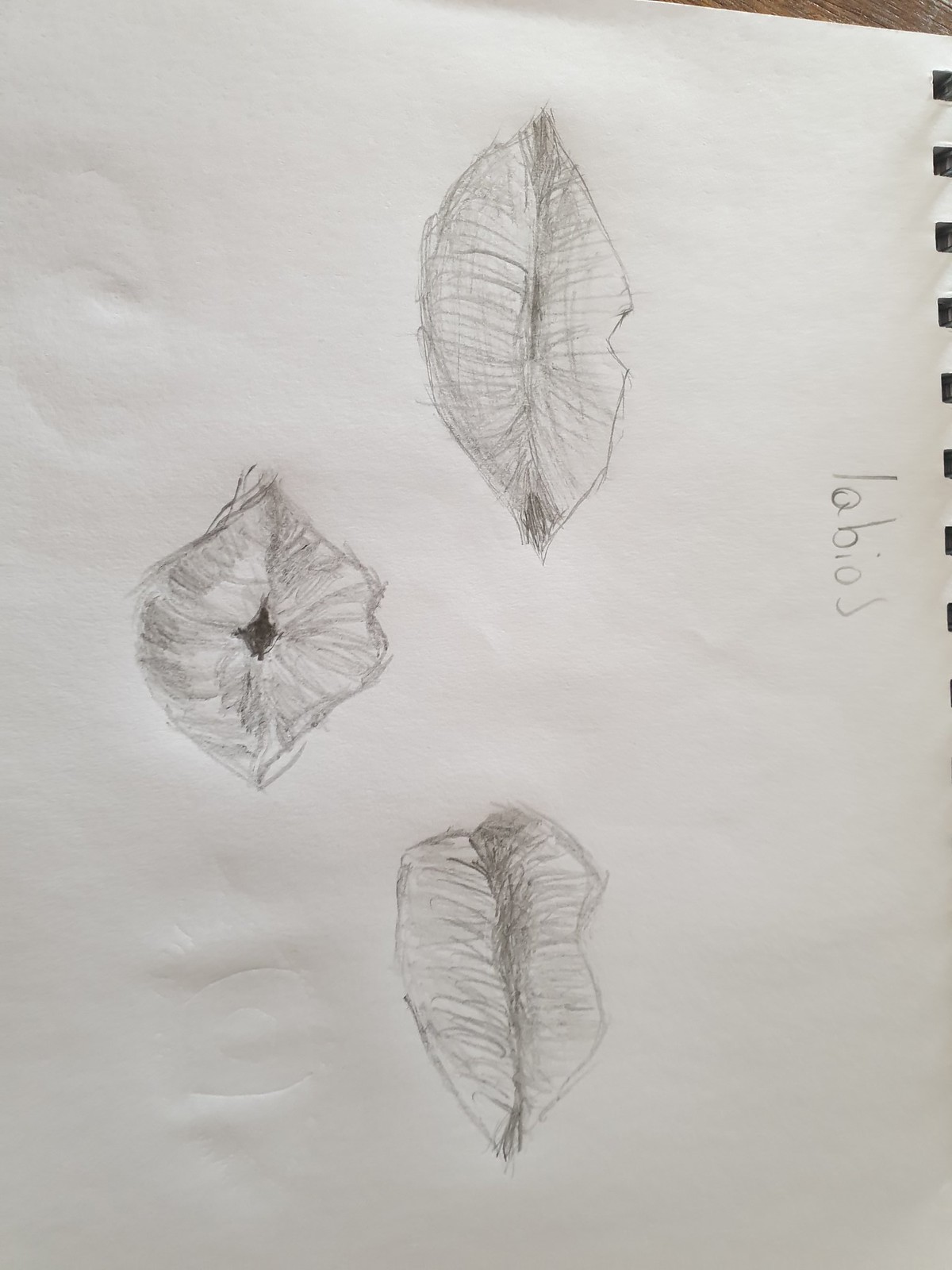The image captures a zoomed-in view of a pencil drawing on what appears to be a sketch pad or notepad, identified by the small square holes running vertically along the right edge. The background in the upper right-hand corner is a beige color, but the specific surface is indistinguishable due to its limited visibility. The photograph is taken at a slanted angle, revealing the Spanish word "labios" (meaning "lips") written in pencil. The drawing features three pairs of lips: two pairs are positioned side by side with the lips closed, while the third pair is depicted with the lips slightly puckered, as if in the act of kissing.